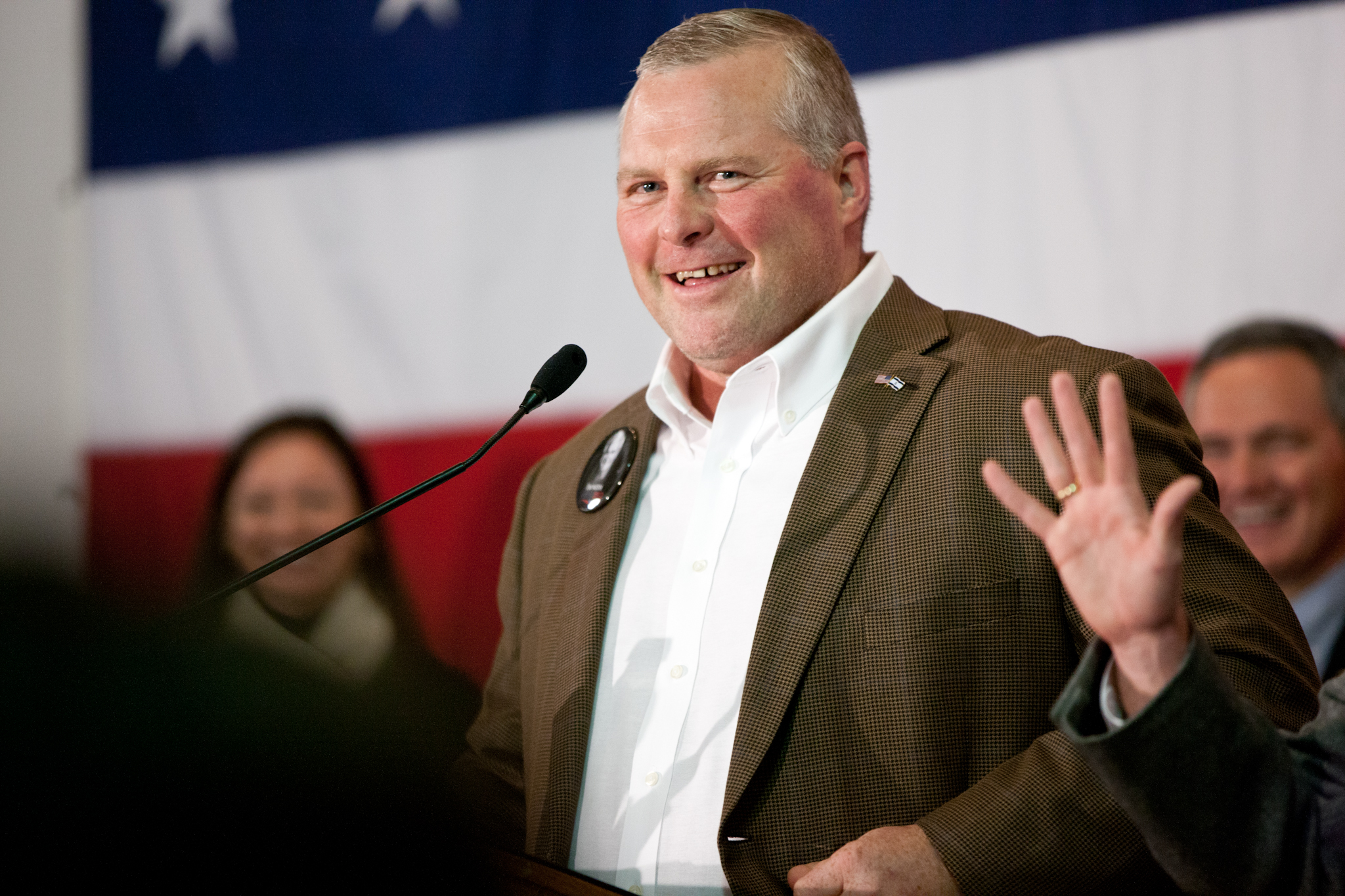The photograph captures a presentation scene where an older, slightly heavier Caucasian man, likely in his early 60s, stands on a stage. He is positioned behind a light brown wooden podium with a slanted top, and a stand microphone is angled towards his mouth. The man is smiling, revealing his top row of teeth, and his ruddy cheeks contribute to his approachable demeanor. His short hair is a mix of brown and gray. He is dressed in a brown business coat with a subtle checkered or diamond-like pattern, which is open, showing a pristine white button-up shirt with the collar buttoned down but the top button undone. A metal pin adorns his right lapel. His right hand rests on the podium while a partially visible hand, adorned with a gold ring, appears in the bottom right corner of the photograph, belonging to another individual. In the background, the American flag casts a patriotic atmosphere with its iconic red, white, and blue colors. Behind the man, two other individuals, one a girl to the left and a guy to the right, smile and add a sense of camaraderie to the scene.